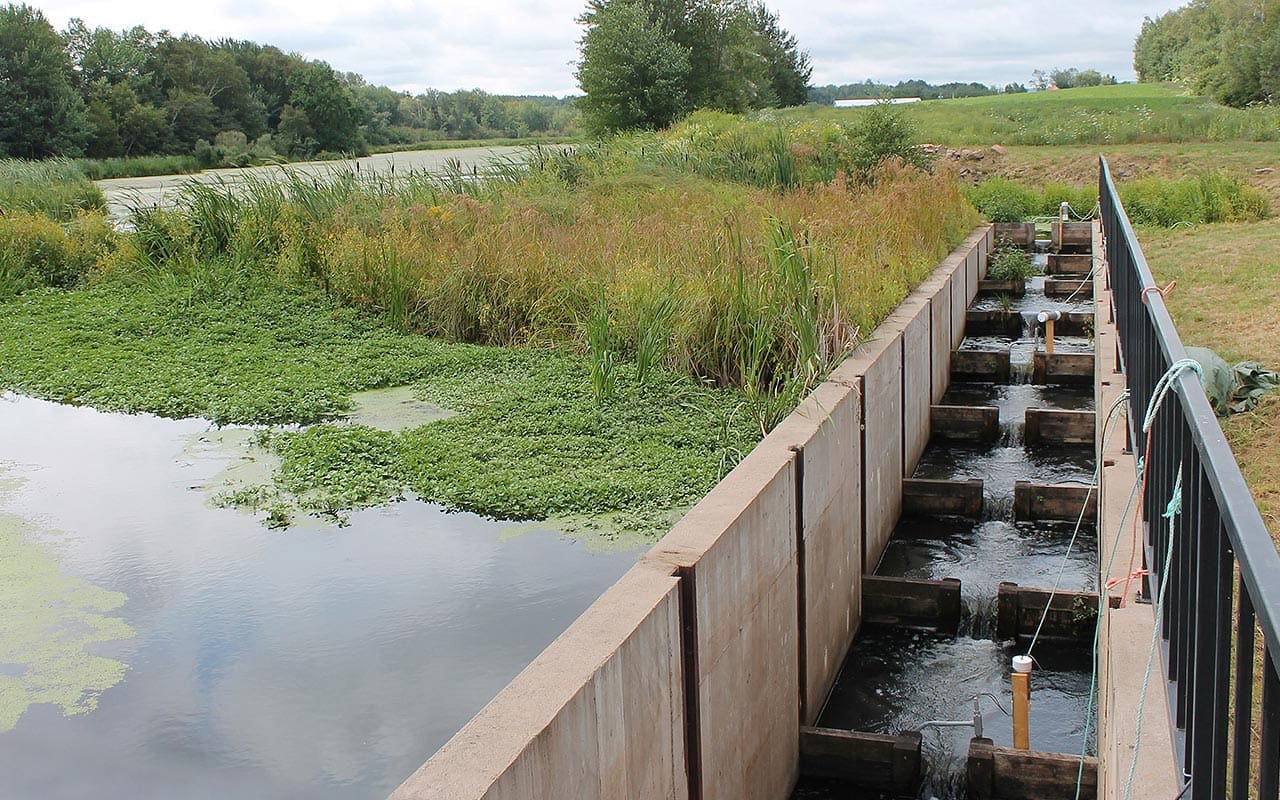This outdoor photograph features a serene natural scene with a river flowing through a lush, grassy field. The river's surface is dotted with floating algae, lily pads, various water plants, and reeds near the banks. Dominating the center of the image, there is a concrete structure resembling a dam or water canal, consisting of two cement walls with evenly spaced notches and square channels. These channels appear to regulate water flow, potentially for flood control or irrigation purposes.

Adjacent to the water, there is some machinery likely used for monitoring and controlling the water pressure and flow rate. The scene extends to show grassy hills and a few scattered flowers, creating a picturesque backdrop. In the distance, a large warehouse stands, presumably used for storing farm equipment like tractors. Trees border the scene, adding to the natural ambiance, while the sky is overcast with clouds, suggesting a cloudy day. The overall setting seems to be a rural area, possibly in China or the United States, characterized by vast grassy fields and an abundance of greenery.